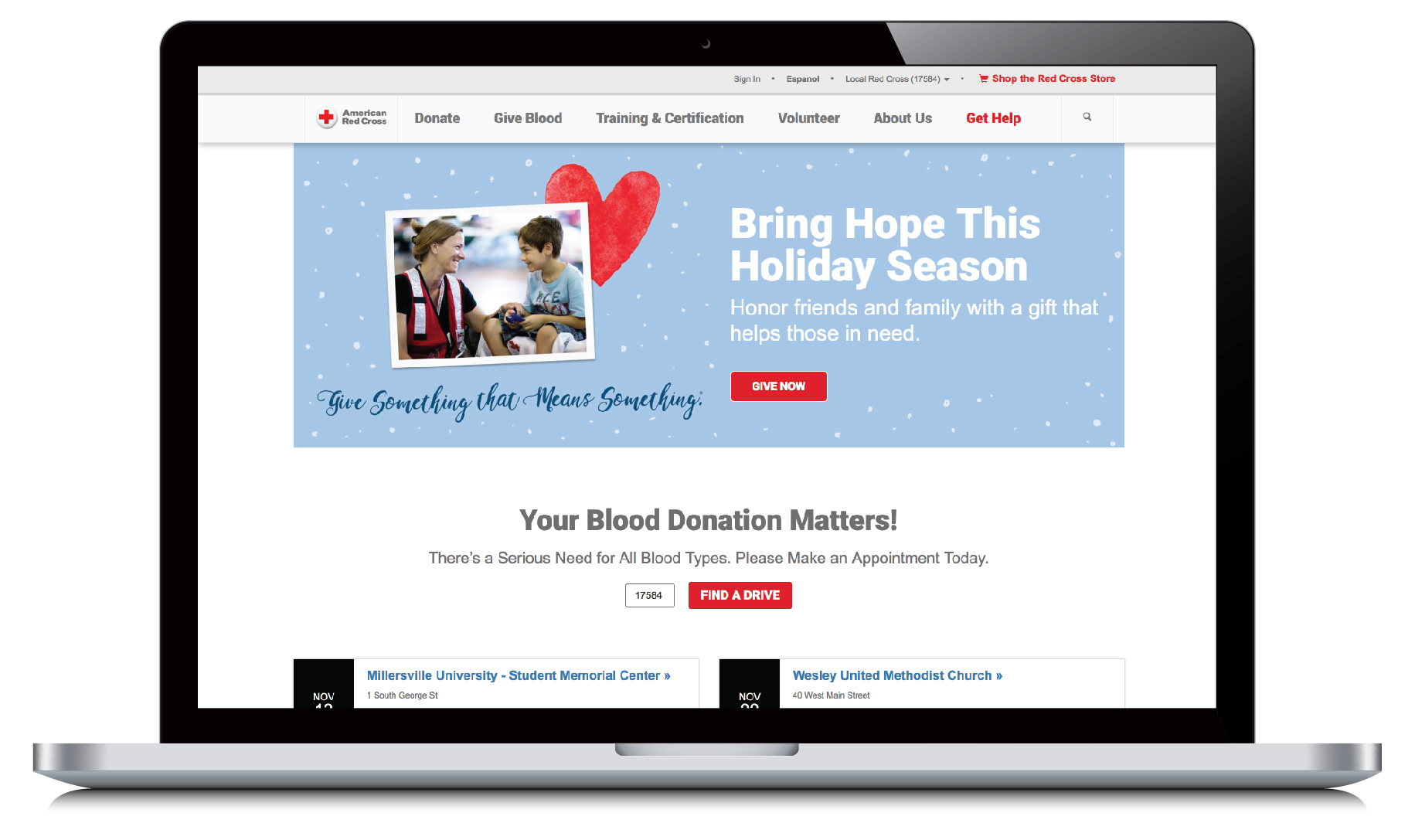The image showcases a laptop with a pristine white background displaying the main webpage of the American Red Cross. The website interface features several primary tabs in the navigation bar: Donate, Give Blood, Training and Certification, Volunteer, About Us, and Get Help, with the 'Get Help' tab highlighted in red font, while the rest are in black. At the top right corner of the screen, there are options for signing in, viewing the site in Español, and accessing local Red Cross store information, as well as a link to Shop the Red Cross Store. A search bar is also prominently visible, allowing users to search the site.

The main section of the webpage contains various thematic headings and prompts. A central banner reads "Bring Hope This Holiday Season," followed by the phrase "Honor Friends and Family with a Gift that Helps Those in Need." Another stylized message in cursive says, "Give Something That Means Something," accompanied by a 'Give Now' button inviting donations. 

Below this, there is a critical appeal stating, "Your blood donation matters. There is a serious need for all blood types. Please make an appointment today." This section includes a 'Find a Drive' button for locating local Red Cross donation events, with specific listings such as the Millersville University Student Memorial Center and Wesley United Methodist Church appearing to announce blood drive events scheduled in November. Additional informative text is discernible beneath this, providing further details on how to participate and contribute.